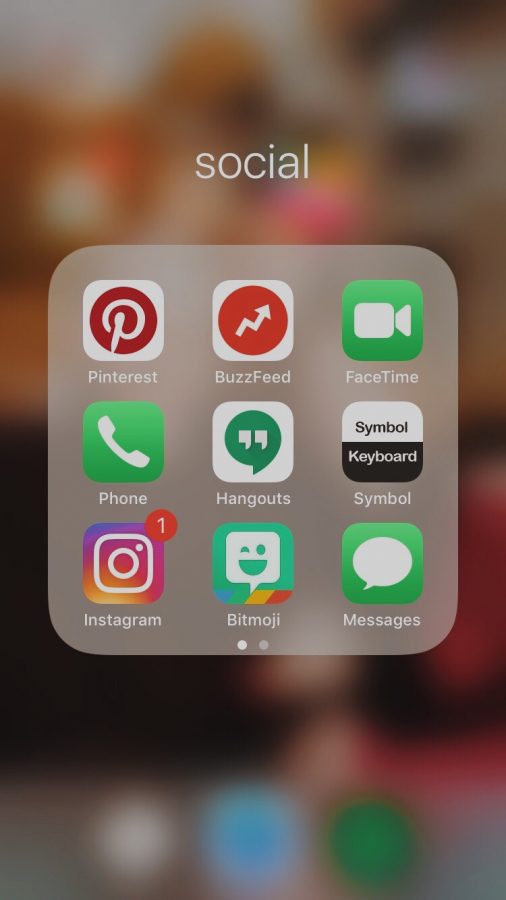The caption describes a screenshot of a smartphone's "Social" folder. Below is a cleaned-up and detailed caption:

---

The screenshot displays a smartphone's "Social" folder. Within this folder, a collection of application icons is neatly arranged inside a rounded rectangle. Visible apps include Pinterest, BuzzFeed, FaceTime, Phone, Google Hangouts, Instagram, Bitmoji, and Messages. Notably, there is a red notification badge with the number "1" on the Instagram icon, indicating a waiting message or notification. The word "socials" is labeled in lowercase white text beneath the folder. The background of the screenshot appears blurry, suggesting the user's focus is on opening the folder and viewing the listed applications. This detailed view captures all elements prominently within the screenshot.

---